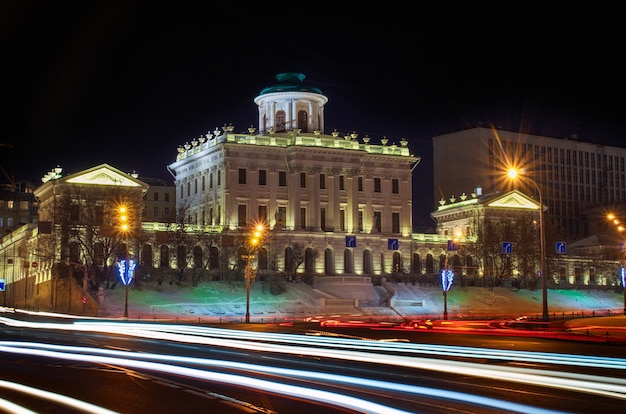This image captures a regal government building centered in a square, illuminated vividly against the night sky. The building, adorned with numerous arches stretching from one side to the other, features a distinguished cupola at its center. In the foreground, a body of water reflects the brightness of the scene, while streaks of white lights on the bottom left hint at the passage of cars, suggesting a time-lapse effect. The scene is painted with an array of colors: white, red, black, and blue, complemented by the presence of several trees and multiple street lamps casting bright rays. Surrounding the main building, other structures are equally lit in various hues, including yellow and blue, contributing to a festive, almost celebratory ambiance, despite the absence of people.